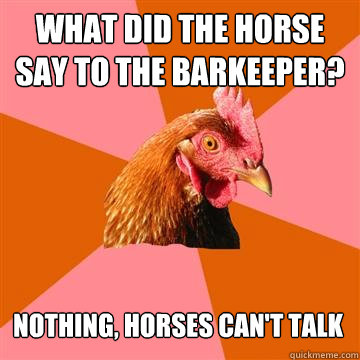The image features a bald, middle-aged man posing provocatively on a bed in a bedroom setting. He is dressed minimally in a black jockstrap or g-string, accentuating his muscular, bare-chested physique. The man is positioned directly in the center of the frame, on his hands and knees, with a large cylindrical object strategically placed to appear as if it's part of his body. He gazes into the camera with a playful smile, exuding a mix of playfulness and seduction. The bed he is on has a mix of textures and colors, including leather black and red pillows, a black and gray army-type bedspread, and brown bedposts. The background includes a gray wall, headboard, visible wall outlets, and light switches, indicating an indoor bedroom environment. The only text in the image is the word "HAI," written at the bottom. The overall color palette of the image comprises gray, brown, black, white, and red.